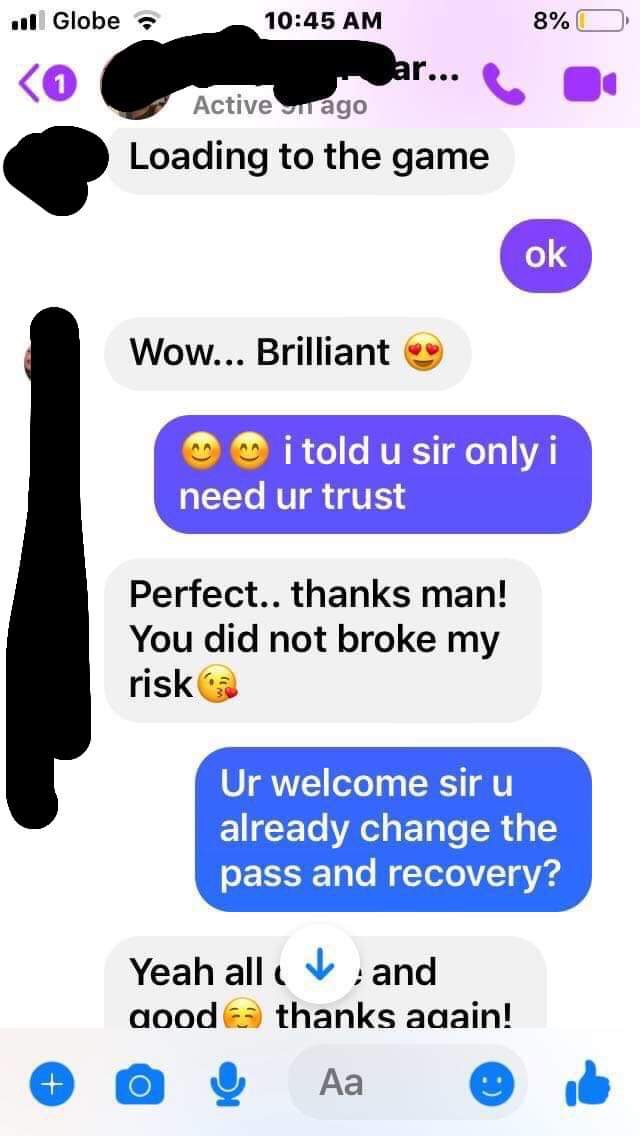This image shows a vertically oriented screenshot of a text message exchange between two people on a smartphone, with some of the names and text details redacted using black ink-like marks, likely done through an editing app. The conversation occurs at 10:45 AM, with the phone displaying an 8% battery and connected to the Globe Network.

The text conversation reads:

1. "Loading to the game."
2. "Okay."
3. "Wow, brilliant 😊❤️."
4. "I told you, sir, only I need your trust."
5. "Perfect... thanks, man. You did not break my wrist! 😘."
6. "You're welcome, sir. You already changed the path of recovery?"
7. "Yeah, all done and good 😊. Thanks again!"

The bottom of the screen includes icons for adding media, such as a plus symbol, a camera, a speakerphone, and a smiley face. The image's edits give it a peculiar appearance, as the redactions seem digitally applied rather than manually marked.